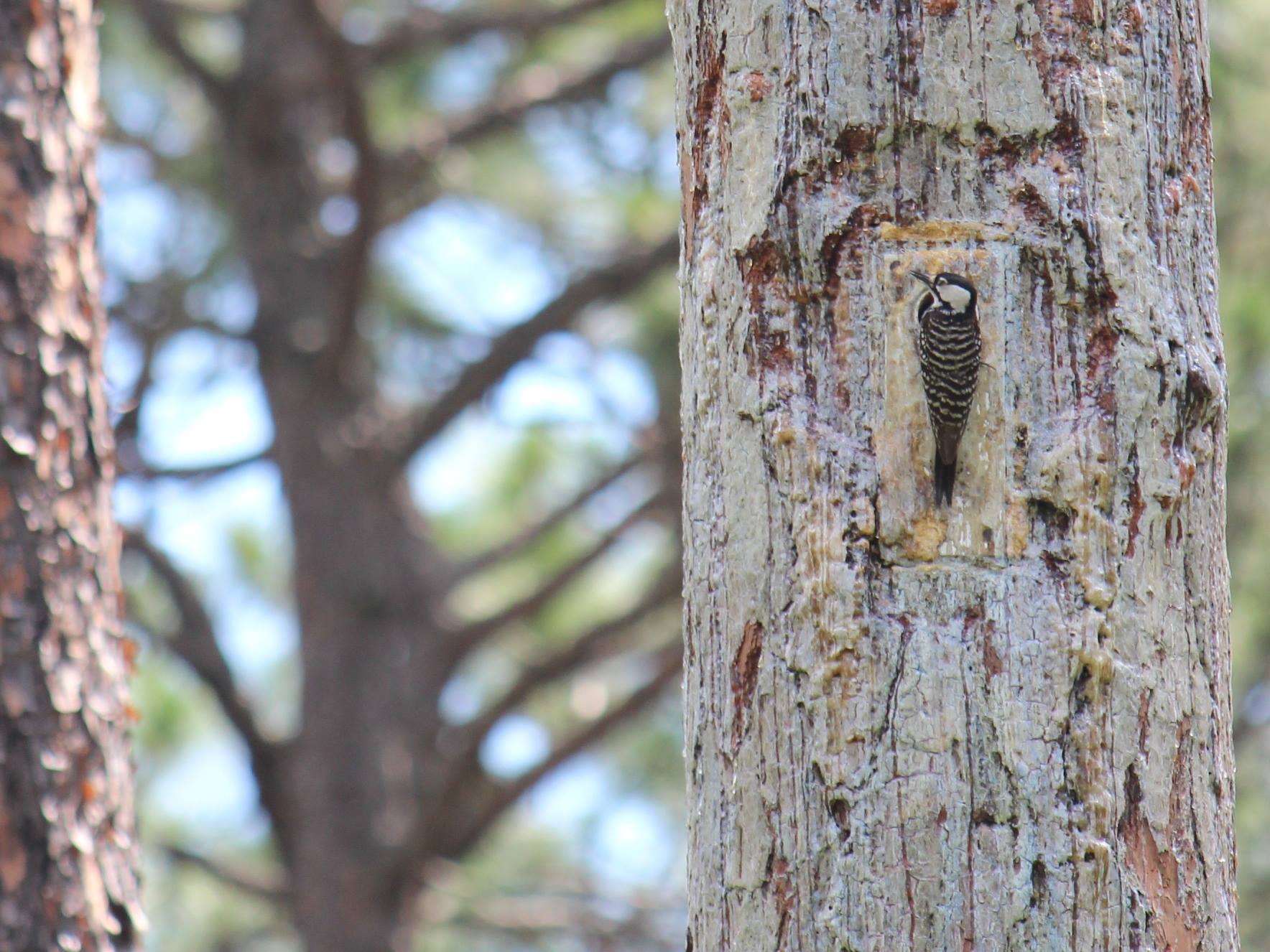This detailed close-up image captures a small black and white striped bird, likely a woodpecker, perched on an old and moldy white tree trunk that stands centrally in the picture. The bird, located right at the middle of the tree, slightly elevated, showcases its distinct markings: a predominantly black body with dark brown patches, interspersed with thin horizontal white stripes, and a white area around its cheek. The bird appears to be investigating or pecking at a hole in the trunk. To the left of the image, there's a contrasting brown-barked tree trunk. The background is beautifully blurred, featuring an unfocused view of another tree, green leaves, and glimpses of blue sky, evoking a serene forest scene. The predominant colors in the image are gray, green, blue, brown, black, and white.